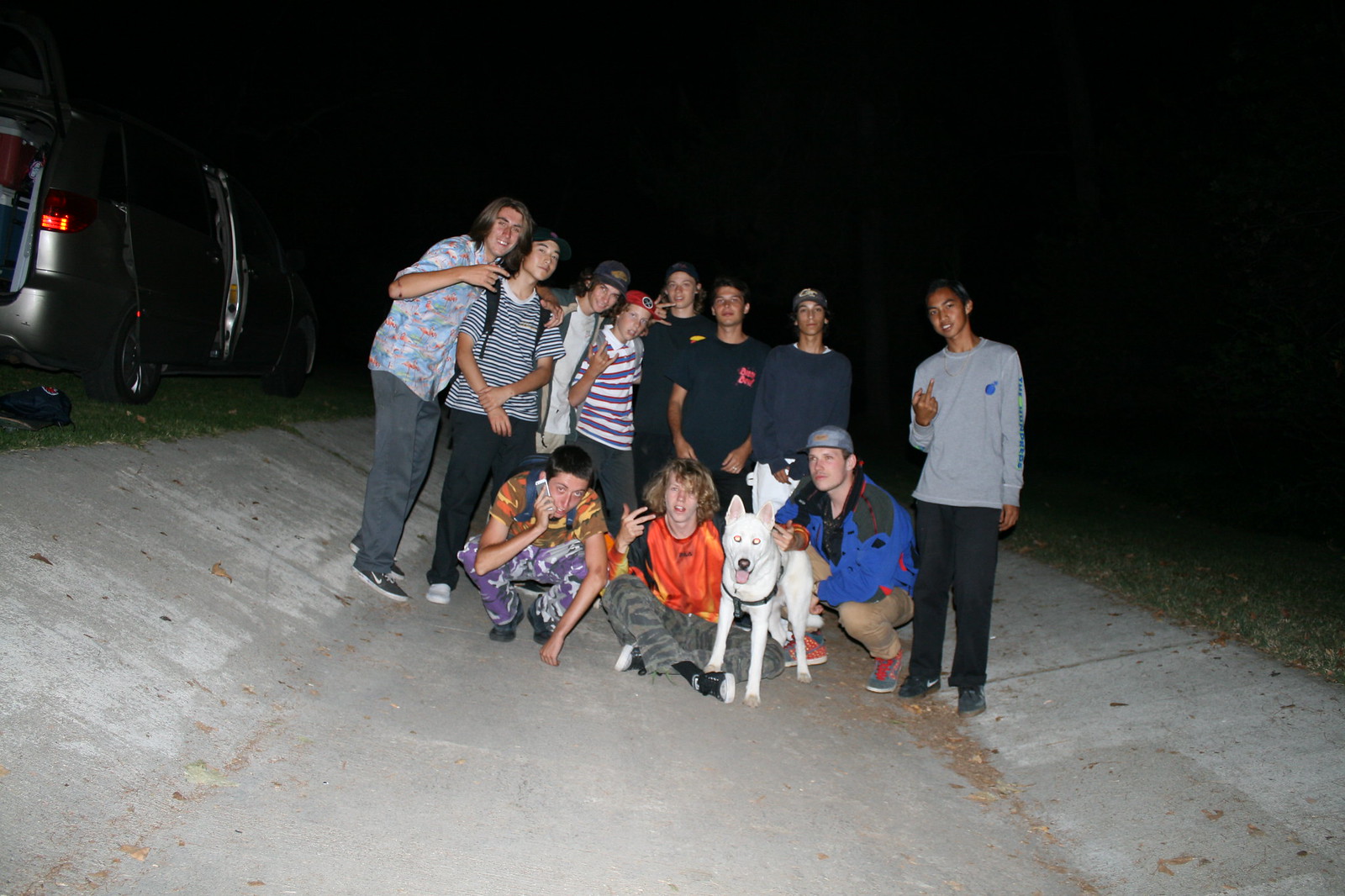This nighttime photograph captures a lively group of 12 young teenage boys posing outdoors on a concrete pathway, with the pitch-black sky behind them. Illuminated by an unseen light source, the boys exhibit an array of playful and casual expressions, making various hand gestures, including one boy on the right, with brown skin and wearing gray shirt and black pants, flipping off the camera. The group appears happy and energetic, with some boys wearing ball caps in red, black, and brown, and a mix of t-shirts in gray, black, orange, purple and white stripes, and black and white stripes. Their pants too vary, including gray, black, tan, and purple camouflage. In the front row, three boys are crouched down, one of whom is absorbed on his cell phone, while another with his arm around a white dog that has a black collar, which is staring directly into the camera. There's a distinctive orange shirt and camo pants worn by one boy, contrasting with another’s tan khaki pants and blue jacket. The left-hand side of the image features an open-door van, indicating they might have paused to take this photo before heading off somewhere. Scattered grass flanks both sides of the otherwise concrete setting, adding to the casual, impromptu feel of the scene.